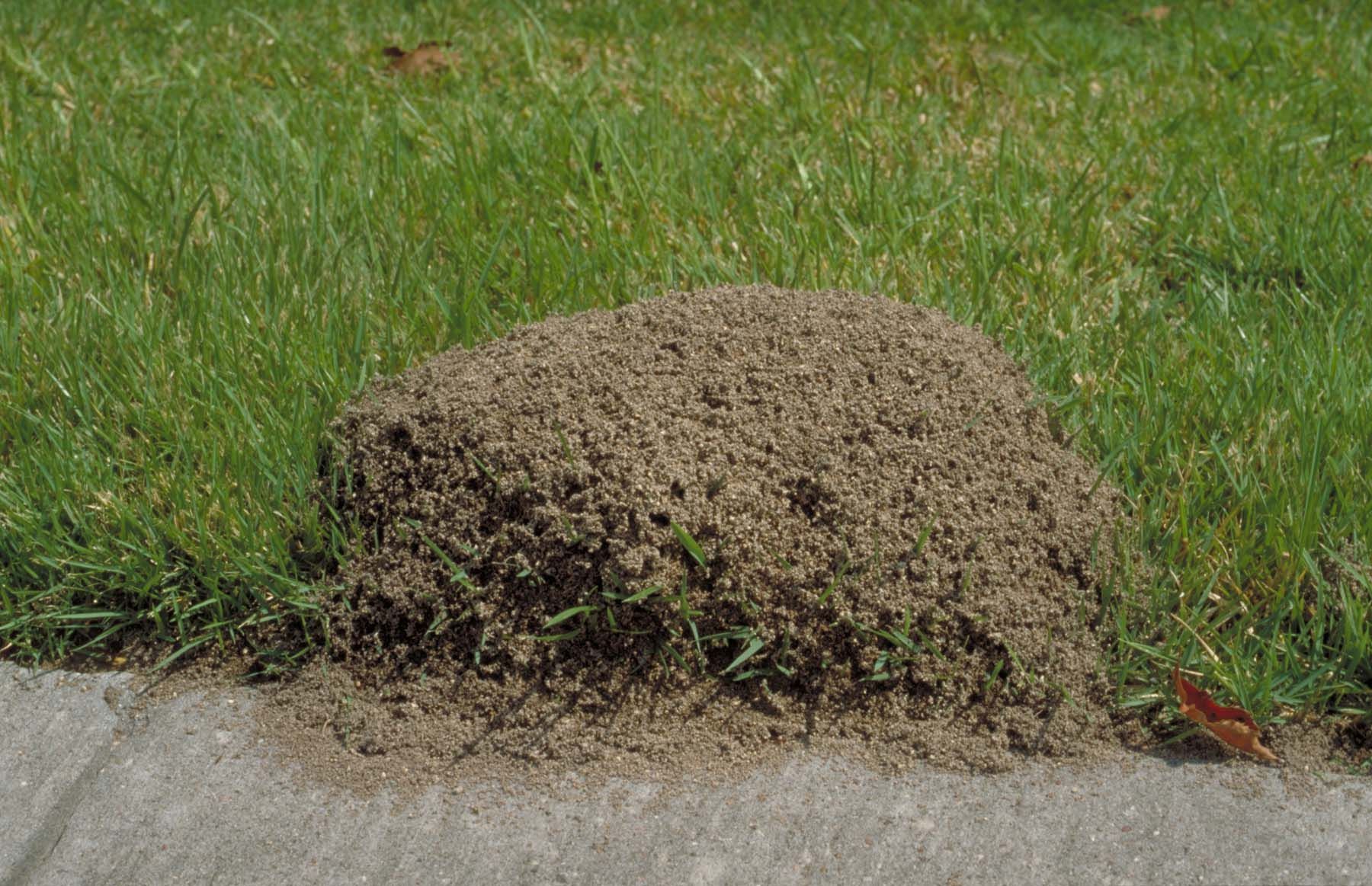The photorealistic image captures a close-up view of a brown, unevenly textured mound of dirt, possibly an anthill, positioned between a gray, paved sidewalk and a patch of green, mown grass. The mound appears to be around five to six inches high and roughly eight inches wide, with parts crumbling onto the sidewalk below. This daytime scene, brightly lit by sunlight, includes small brownish dead leaves scattered near the base of the mound and among the vivid green blades of grass. The setting suggests a yard or park area where the presence of the mound might not be welcomed.